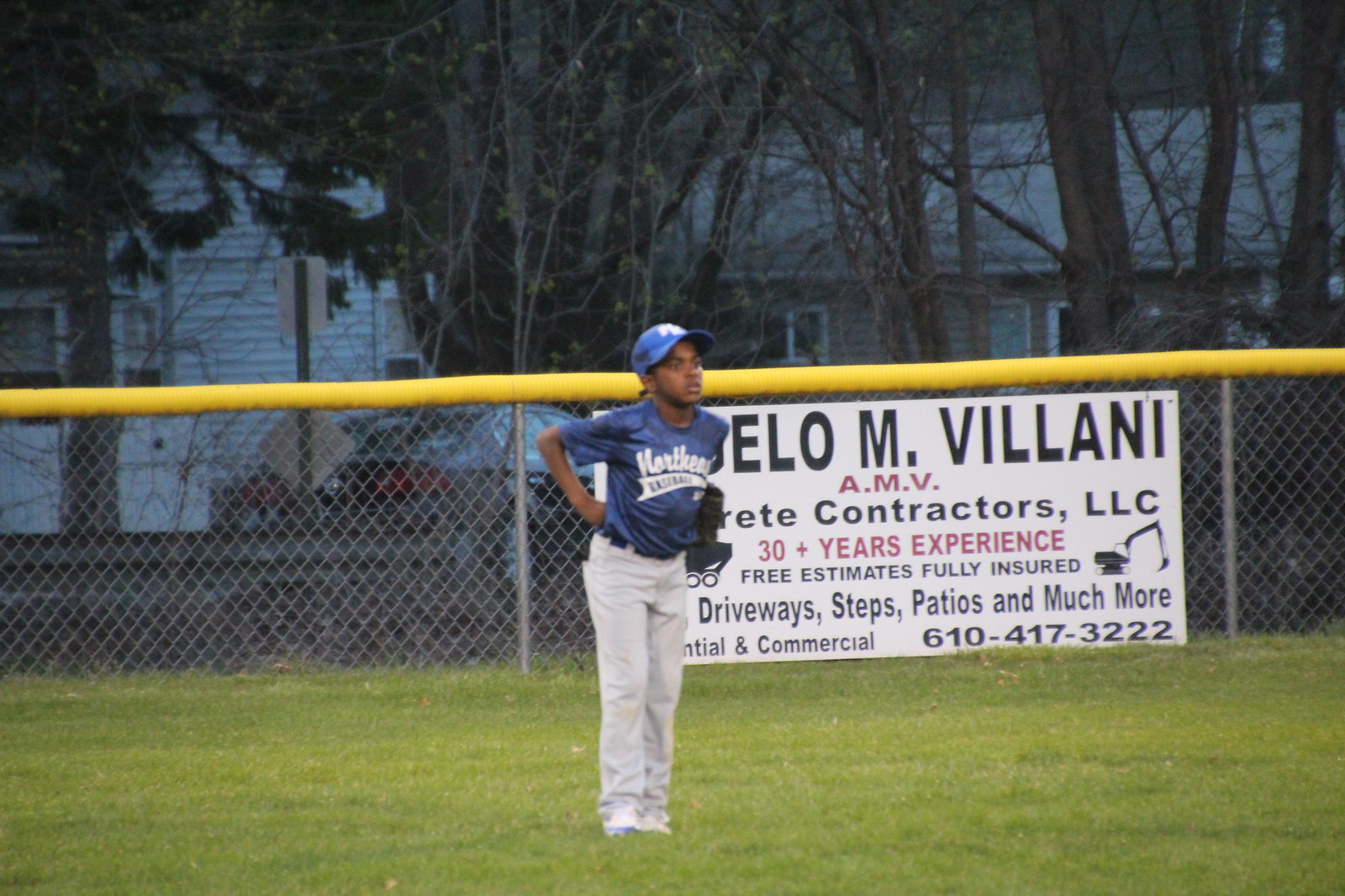A young boy, likely participating in a Little League baseball game, is standing in the outfield of a community baseball field. He wears a blue baseball cap, a blue short-sleeved shirt with "Northeast" written in white, a black belt, and white pants, and he holds a black glove in his left hand. The background features a chain-link fence topped with a bright yellow protective barrier. Behind the boy, there's a sponsor sign for Villani AMV Concrete Contractors LLC, advertising 30-plus years of experience, free estimates, and full insurance, serving both residential and commercial needs, including driveways, steps, and patios. A partial phone number, starting with 617, and various elements such as trees, parked cars, and a glimpse of houses behind the fence complete the scene, indicating a typical suburban neighborhood setting.